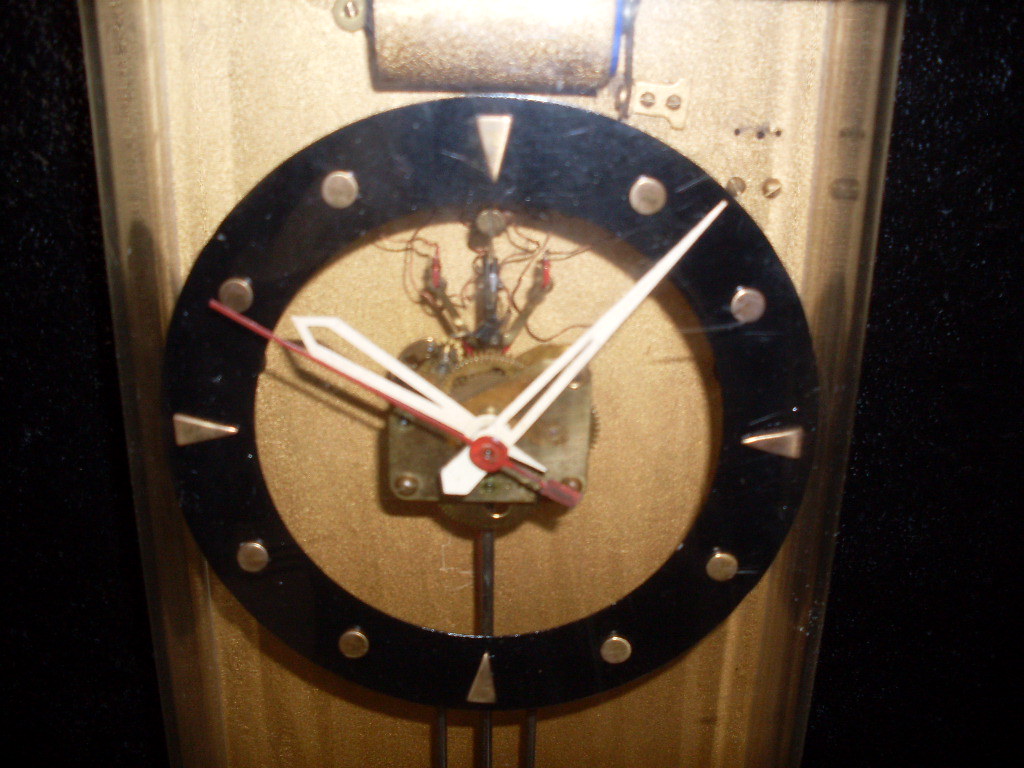This square-shaped image features an elegant timepiece centered against a golden backdrop. The clock itself is circular, enclosed by a thin black border adorned with minimalist dot markers in place of traditional numbers. Bronze triangles accentuate the cardinal points of the circle—top, bottom, left, and right—adding a geometric flair to the design. The clock's hands, distinct in their coloring, include one in white and the other in red, offering a vibrant contrast to the bronze and black elements. The overall aesthetic combines modern minimalism with a touch of classic elegance, highlighted by the rich golden background.